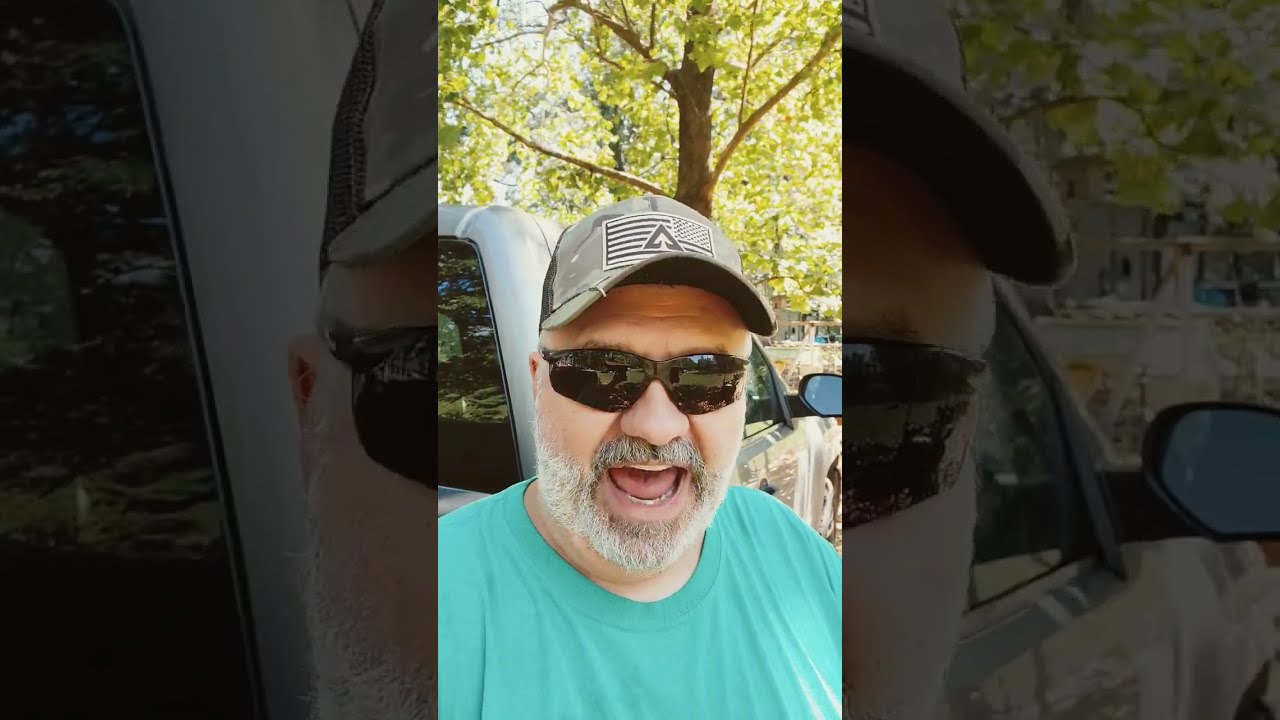This three-panel image features a middle-aged man with a predominantly gray beard, a baseball cap with an unidentified symbol, and large, dark sunglasses. He is wearing a turquoise t-shirt and appears somewhat overweight. The central panel portrays the man with his mouth wide open, standing in front of a gray pickup truck with tinted windows. A large, leafy tree is prominently visible behind the truck, and traces of grass and possibly a distant building are discernable in the far right corner.

The left and right panels are close-up, underexposed blow-ups of the respective sides of the man's face from the central image. These panels magnify portions of his sunglasses, cap, and the truck, creating a darker and more opaque effect. The composition suggests an artistic approach, emphasizing detailed fragments of the main photograph through its elongated format and distinct cropping.